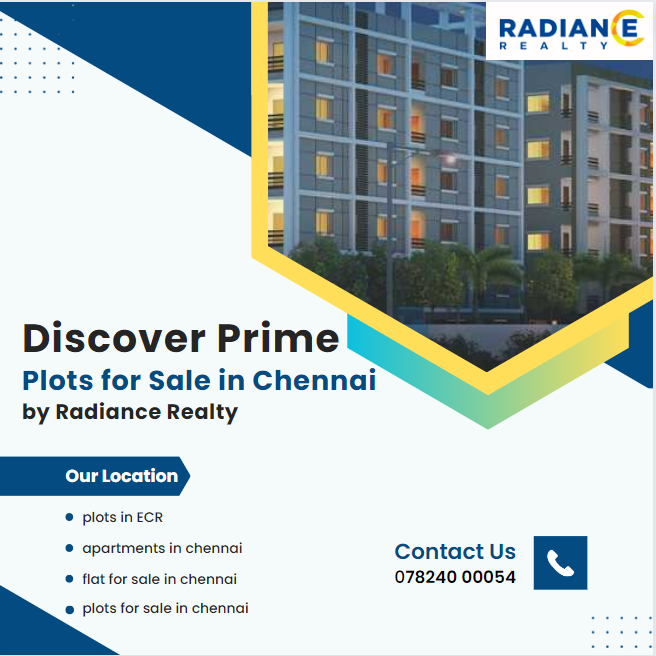This image features an advertisement for Radiance Realty. The top right corner displays their logo, "Radiance Realty," alongside a photograph of a large, multi-story, grey apartment building with numerous windows. Below the building, lush green trees are visible, and a light bulb icon is also present.

In the middle of the left side of the advertisement, bold black letters declare "Discover Prime." Below this, blue text reads, "Plots for Sale in Chennai," and smaller black letters indicate the offering is "By Radiance Realty." Further down, within a blue rectangle, the words "Our Location" are written in white. Beneath this section are four bullet points listed in blue, detailing: plots and ECR apartments in Chennai, flats for sale in Chennai, and plots for sale in Chennai.

On the lower right side, the caption "Contact Us" appears next to an image of a telephone handset, with the accompanying phone number: 078-240-00054.